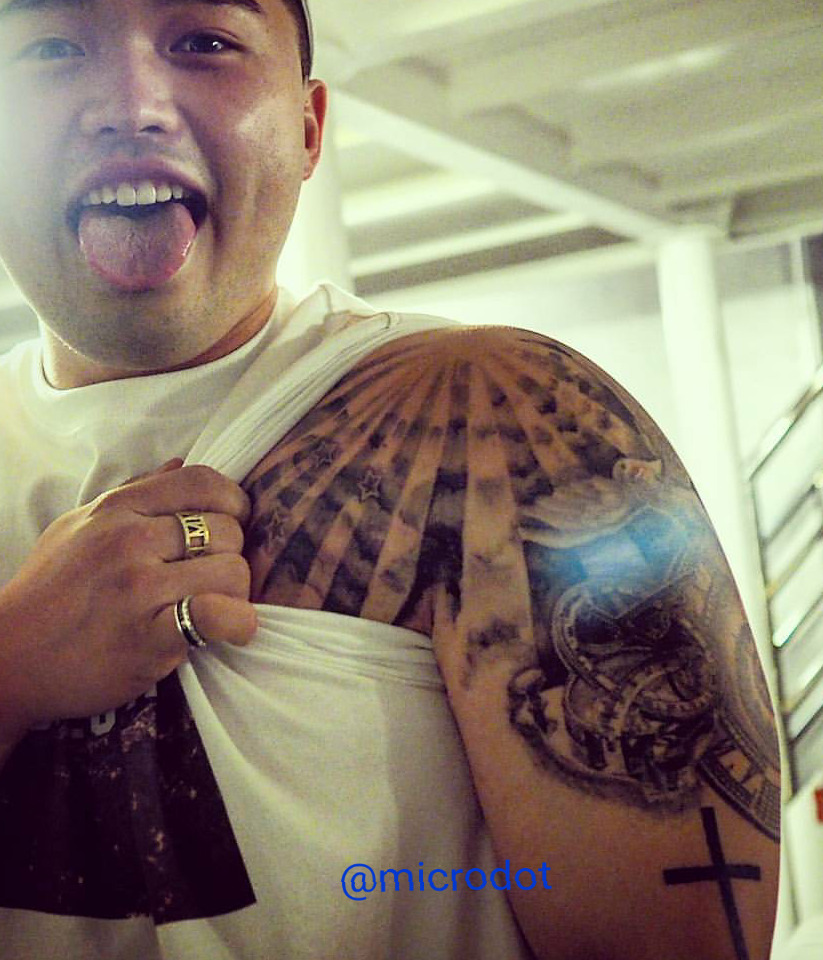This indoor photograph captures an Asian man with very short hair, wearing a white t-shirt, sticking his tongue out playfully. He is using his right hand, adorned with a gold and a silver ring, to lift the left sleeve of his t-shirt, revealing an elaborate black tattoo on his upper arm and shoulder. The tattoo features a cross above the elbow and extends upwards, designed with sun rays and a small squirrel-like figure, showcasing intricate black and gray shading. The background reveals a white-painted interior with a ceiling supported by white poles and a staircase visible. At the bottom of the image, blue text reads "@micro dot."